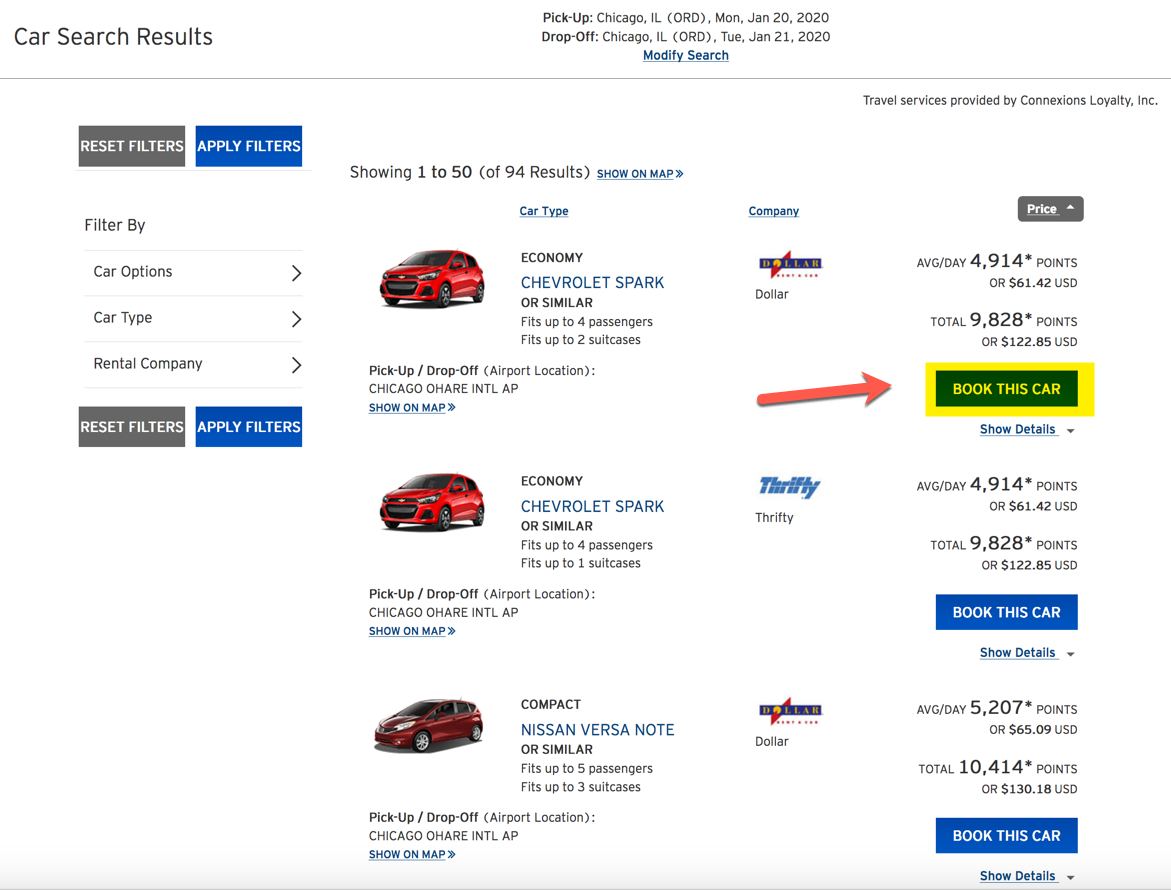Screenshot of Car Search Results Page

In the upper-left corner, there's a section labeled "Car Search Results" presented on a white background. 

On the right side, in the middle of the screen, the pickup and drop-off details are displayed. The pickup point is listed as Chicago, Illinois (ORD) on Monday, January 20, 2020, and the drop-off point is Chicago, Illinois (ORD) on Tuesday, January 21, 2020. Below this section, there's a hyperlink labeled "Modify Search."

On the left-hand side of the page, there are options to "Reset Filters" and "Apply Filters," enclosed in dark gray and blue rectangles, respectively. Further below, there are three filtering options: "Car Options," "Car Type," and "Rental Company." There are also buttons for resetting and applying filters again.

To the right side of the filtering options, it states "Showing 1 to 50 of 94 results," with an additional hyperlink that says "Show on Map."

The first car listing is an economy vehicle, specifically a Chevrolet Spark or a similar model. This car can accommodate up to four passengers and fit up to two suitcases. To the right of this specification, the rental company is identified as Dollar. The pricing details mention an average daily rate of 4,914 points or $61.42 USD, with a total cost of 9,828 points or $122.85 USD for the rental period.

Lastly, there is an option to book this car, highlighted in a yellow rectangle with a right arrow pointing to it.